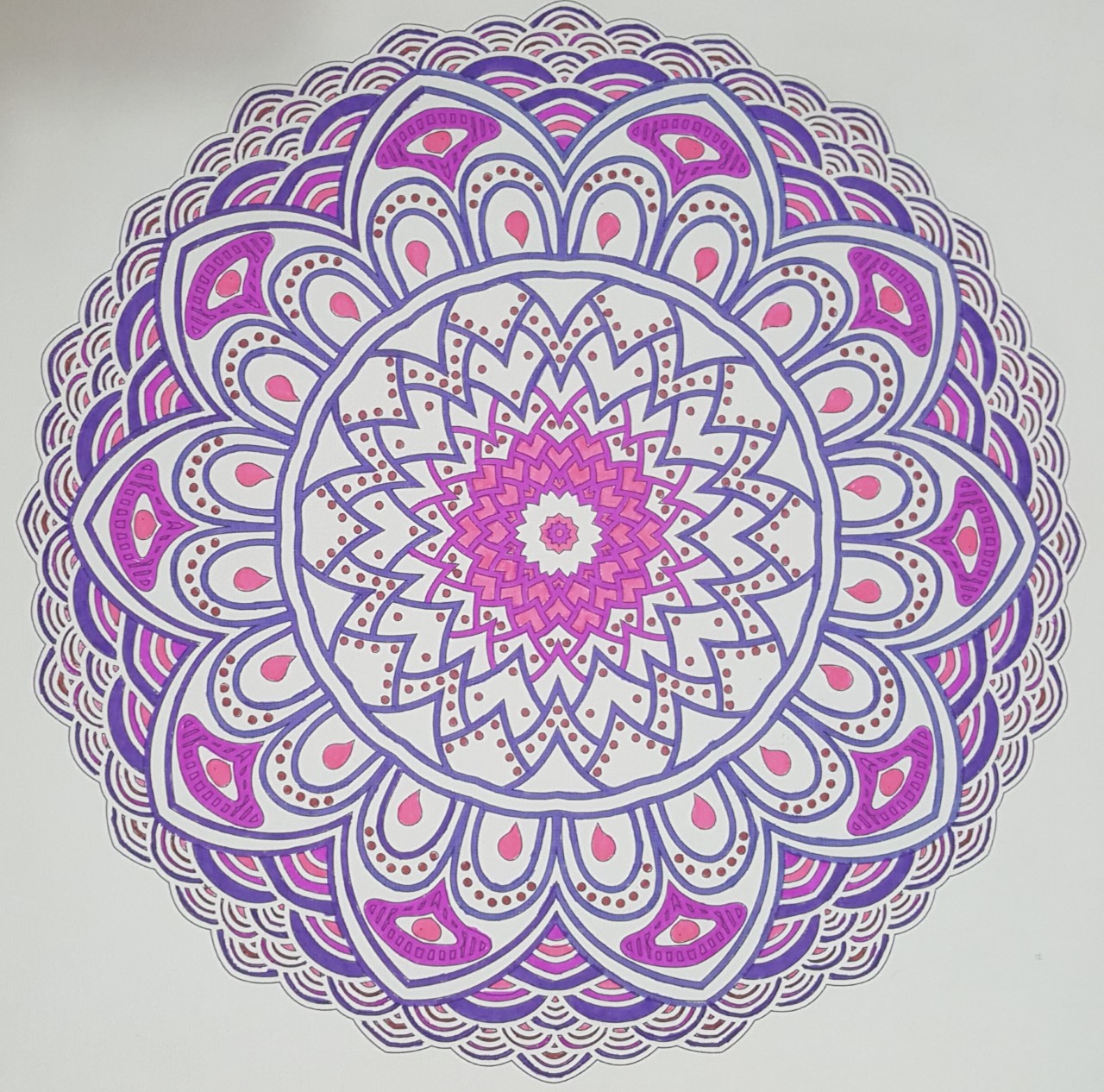This image depicts a meticulously detailed mandala, exhibiting a spiritual and intricate design reminiscent of Indian artistry. The mandala resembles a large flower, with numerous layers of petals radiating outward from a central point. The artwork appears to be hand-drawn, likely using markers, on a piece of white paper, as suggested by the slightly irregular line work. 

The predominant color is a rich purplish-blue, which outlines the circles and petals, providing a bold framework for the design. Within these outlines, the details are highlighted in vibrant shades of light purple and lighter pink, bringing a dynamic contrast to the piece. Additionally, small dots in a reddish-brownish-orange hue are scattered throughout, adding an extra layer of intricacy.

The mandala consists of three distinct layers. The core layer is dominated by pink and purple tones, creating a warm and inviting center. Moving outward, the colors alternate between blue and white, creating a visually appealing pattern. The overall effect is a harmonious blend of colors and shapes, capturing the essence of traditional mandala art while showcasing the unique character of the hand-drawn medium.